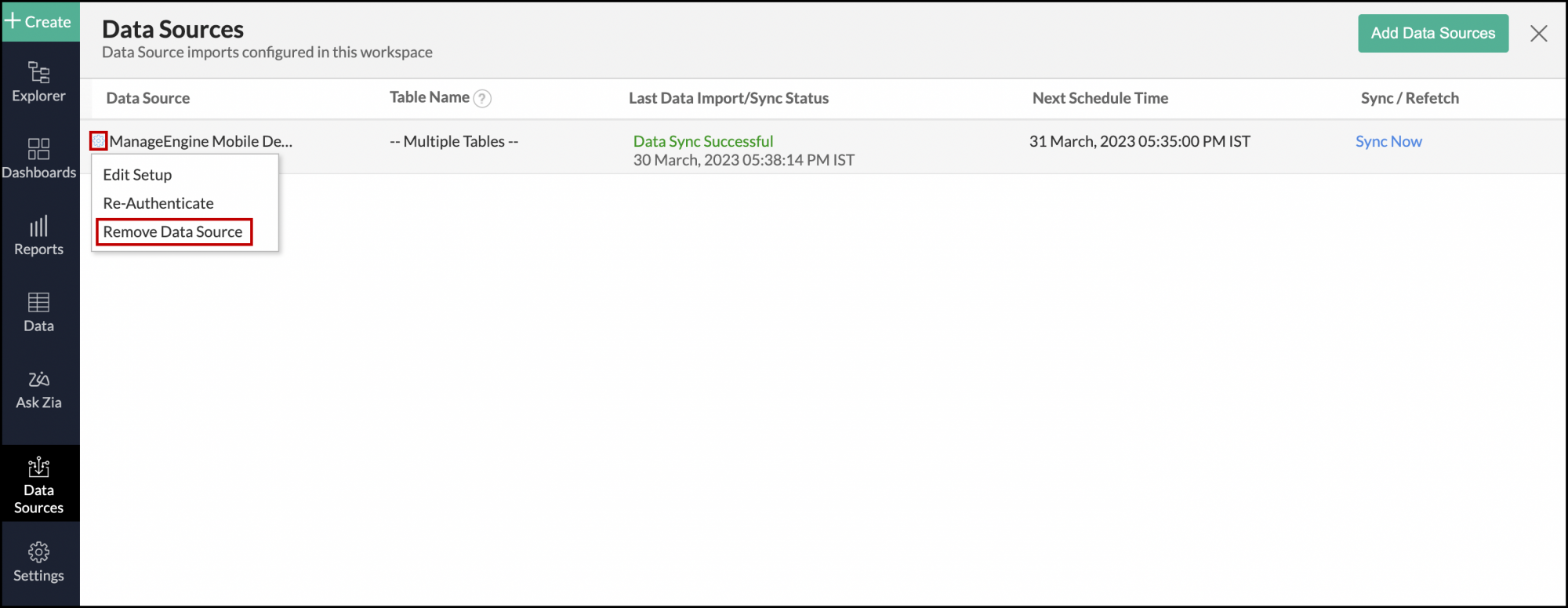The computer window displayed is titled "Data Sources," prominently written in black against a gray bar at the top. Just beneath the title, in smaller text, it reads "Data Source Imports Configured in this Workspace." On the far right side of the header bar, there is a green button labeled "Add Data Sources."

To the left side of the window, there's a vertical black bar featuring a series of options arranged vertically: a green button at the very top labeled "Create," followed by "Explore," "Cyber Ads," "Reports," "Data," "Ask," and "Data Settings."

The main body of the window presents detailed information about a specific data source named "Manage Engine Mobile Device," which is prominently marked and highlighted in red. The information is organized into four additional columns labeled "Table Name," "Last Data Import," "Sync Status," "Next Scheduled Time," and "Sync Refresh."